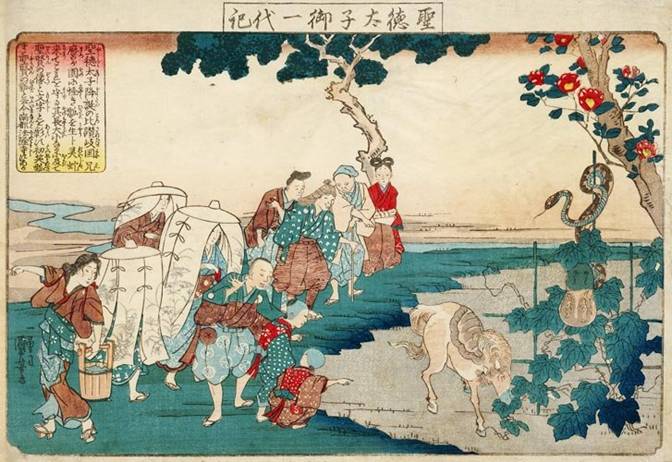The image is an intricate ukiyo-e style Japanese painting set in an outdoor scenery with vibrant green grass and a variety of lush trees. On the right-hand side, a prominent tree adorned with red and yellow flowers extends into the upper corner, while blue-leaved trees add a cool hue to the composition. Near the middle stands another tree, and among the leaves, a snake ominously looks down, seemingly preparing to strike. The central focus shows a white horse, its head lowered as if drinking from a nearby body of water or munching on blue leaves. 

To the left of the horse, there is a lively group of people dressed in traditional Chinese attire, their expressions ranging from amusement to curiosity as they point towards the horse. The children, especially, appear fascinated by the scene. Chinese writing, set against a gradient backdrop of red at the top fading into yellow at the bottom, decorates the upper left corner of the image, adding a cultural touch. The harmonious blend of colors, including blue, red, and yellow, enhances the serene yet dynamic atmosphere of this classic painting.